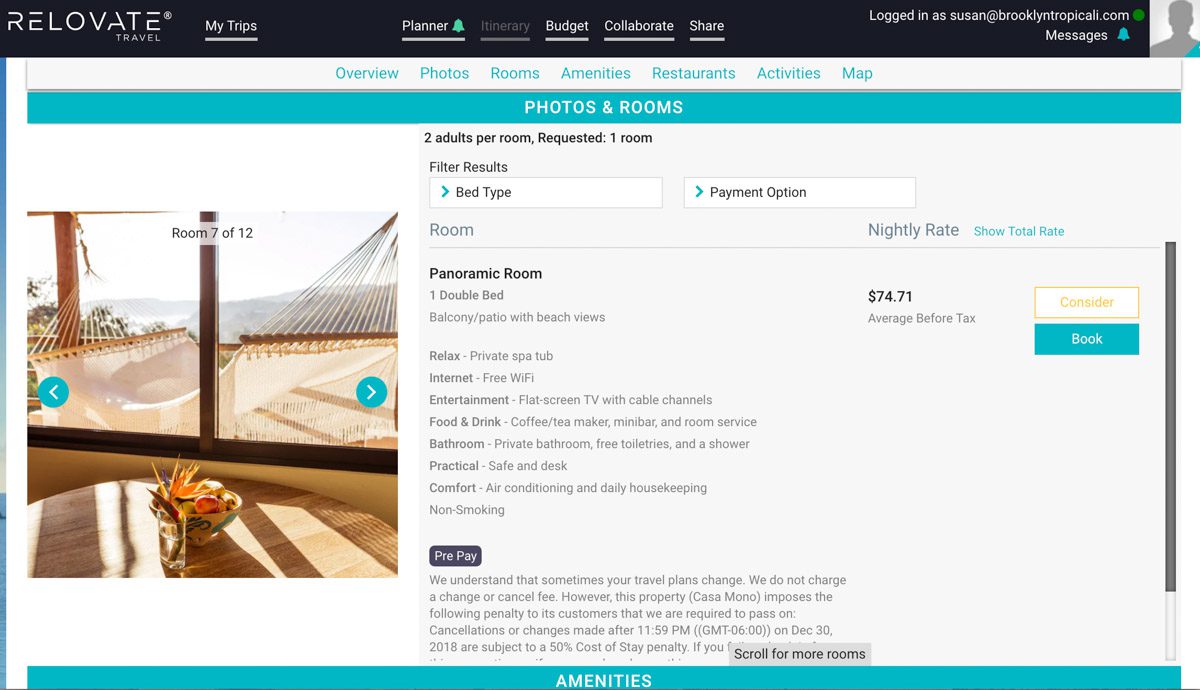In the provided screenshot of the “Relevate Travel” platform, users are greeted with a variety of navigation options: My Trips, Planner, Itinerary, Budget, Collaborate, and Share. The user is currently logged in as Susan at BrooklynNewYorkTropical.com. A message icon is also visible on the screen.

The screenshot features a captivating image of a hammock on a balcony, offering a serene view of a nearby mountain and a table, suggesting a peaceful retreat.

The top menu bar includes tabs for Overview, Photos, Rooms, Amenities, Restaurants, Activities, and Map, highlighting various aspects of the travel experience. In the “Rooms” section, it is noted that two adults have requested one room, with options to filter results by bed type.

The highlighted accommodation is a panoramic room featuring one double bed, a balcony patio with beach views, and a relaxed private spa tub. Additional amenities include internet (free Wi-Fi), entertainment options (a flat-screen TV with cable channels), and food and drink facilities (a coffee and tea maker, mini bar, and room service).

The room boasts private bathrooms equipped with free toiletries and a shower. For practical needs, a safe and desk are available. Comfort features include air conditioning and daily housekeeping. The room is non-smoking. The total cost of the stay is $74.71.